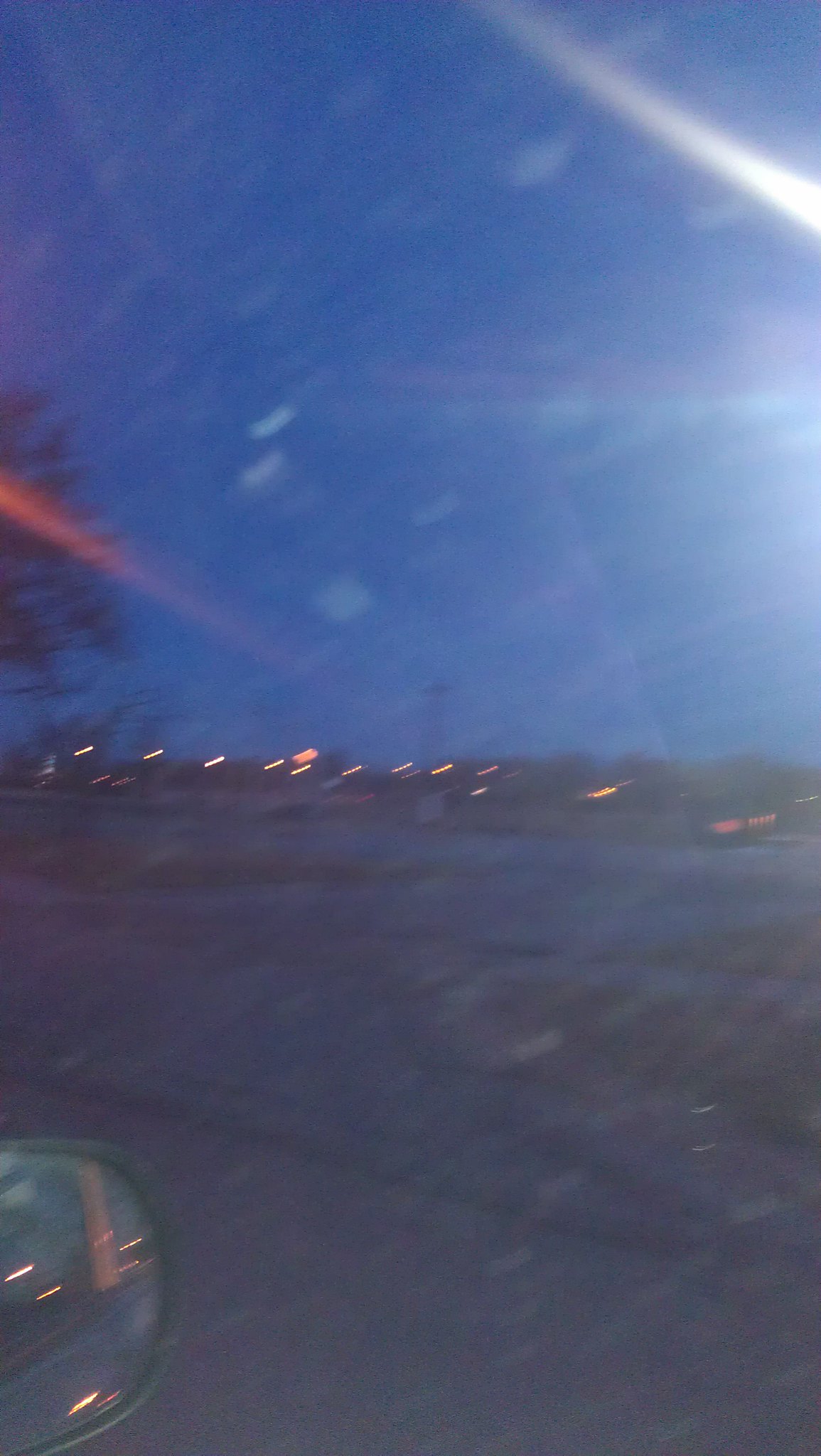An outdoor evening scene captured from a moving vehicle, showcasing a deep blue dusk sky. The image is blurred, characteristic of motion, and there's visible dirt on the window through which the photo was taken. At the bottom left corner, the rearview mirror with a dark housing reflects yellow lights, creating a ghostly white effect on the window. The ground outside appears very dark with a few discernible bumps and hills, offering a hint of uneven terrain. The upper left part of the image reveals the top of a dark-colored tree. Despite an area of yellow and white light ahead visible through the window, the details remain indistinguishable, adding to the mysterious ambiance of the scene.